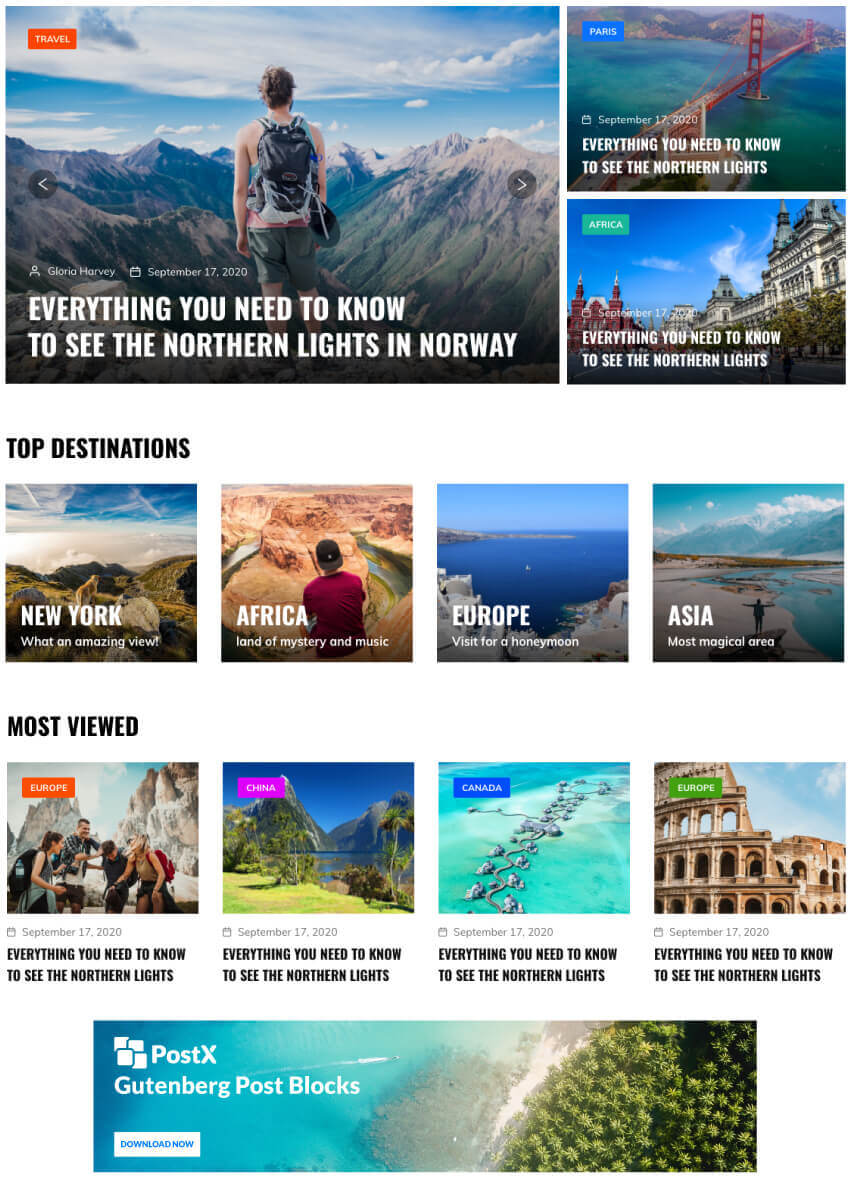Sure, here’s a cleaned-up and highly descriptive caption for the image:

---

The travel page is divided into four distinct sections, with visually engaging arrangements:

**First Section:**
This section features three images where the largest image dominates the left side, occupying more than half of the available space. The image on the left showcases a man standing on a cliff, overlooking a breathtaking mountain range. The man is equipped with a backpack and is dressed in a tank top. Overlaid on this image is a red rectangular box with the word "Travel" inscribed inside it. In addition, there are navigational arrows to the right and left enclosed in a gray circle, suggesting potential navigation through a slideshow. The image's caption reads, "Everything you need to know to see the Northern Lights in Norway."

To the right, there are two smaller images stacked vertically. The top image features the Golden Gate Bridge with a caption that misleadingly reads "Paris" alongside "Everything you need to know to see the Northern Lights." The bottom image presents a scenic view of Lisbon but is incorrectly labeled as "Africa," accompanied by the identical caption, "Everything you need to know to see the Northern Lights."

**Second Section:**
Titled "Top Destinations," this section presents four equally sized images with corresponding captions. The destinations include:
- New York: Accompanied by the enthusiastic caption "What an amazing view."
- Africa: Described as the "Land of mystery and music."
- Europe: Marketed for romance with the tagline "Visit for a honeymoon."
- Asia: Branded as the "Most magical area."

Each destination is visually distinct with unique images representing them.

**Third Section:**
Labeled "Most Viewed," this section contains four options as well, although the specific details and captions for these images are not provided.

---

This detailed caption describes the visual layout, the content of each image, and the text associated with them, providing a clear picture of the travel page's structure and features.